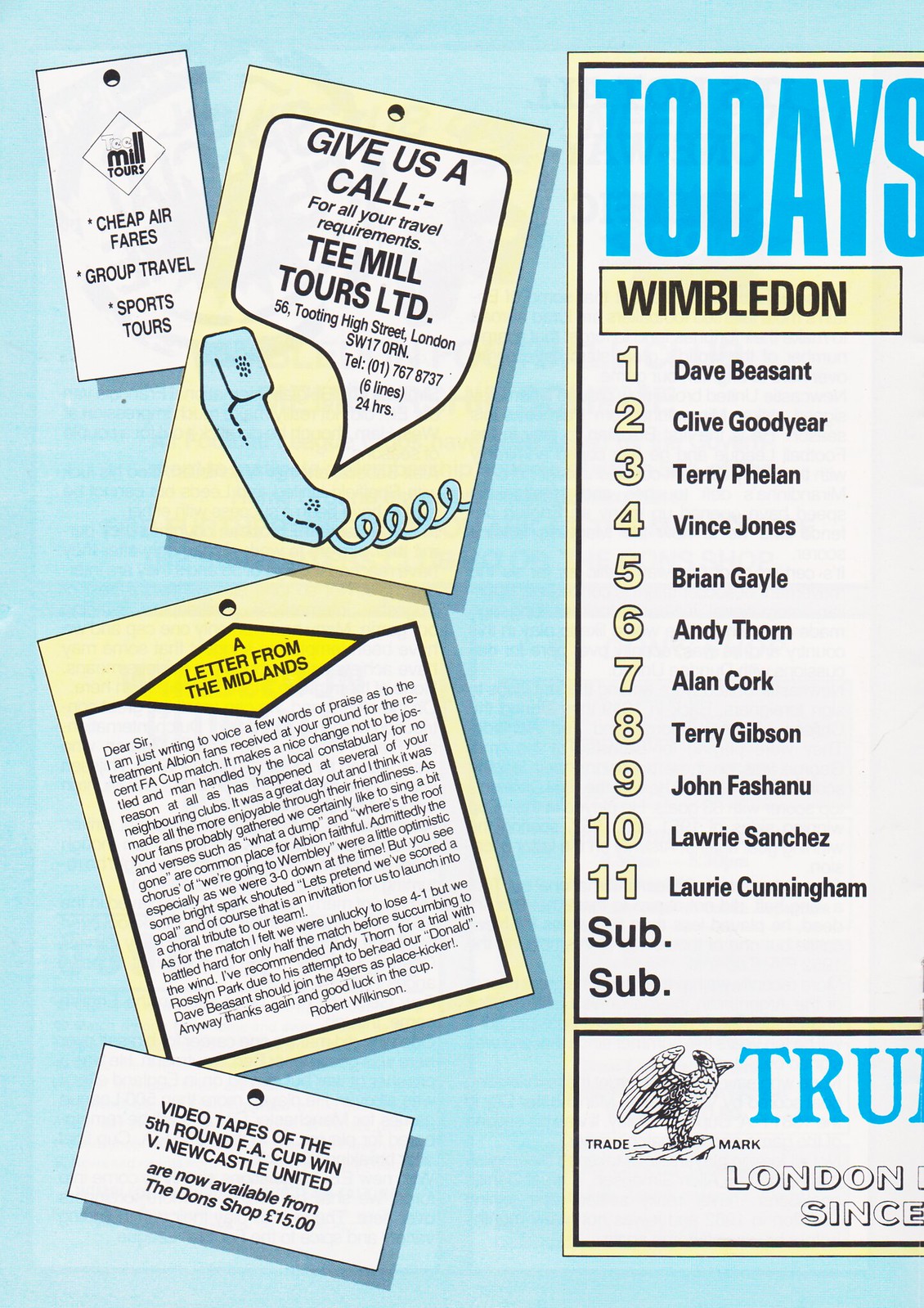This detailed image captures a travel advertisement primarily promoting trips to the UK with a prominent focus on Wimbledon. The right-third of the image is dominated by a vertical, light yellow box. At the top right, in bold blue block letters, it reads "Today's Wimbledon," followed by the names of the 11 players: Dave Besant, Clive Goodyear, Terry Phelan, Vince Jones, Brian Gale, Andy Thorne, Alan Cork, Terry Gibson, John Faschnow, Laurie Sanchez, and Laurie Cunningham. Underneath, yellow numbers enumerate these names.

The left-third of the image, set against a light blue, almost baby blue background, features four images styled as travel tags pinned onto the page. These tags advertise various travel services such as "Cheap Airfares, Group Travel, Sports Tours," accompanied by a call-to-action: "Give us a call for all your travel requirements." It lists "T-Mail Tours Limited, 56 Hooting Street, London, SW 17 ORN, telephone 017678737, six lines, 24 hours."

Another tag promotes videotapes of the fifth-round FA Cup win against Newcastle United, priced at 15 pounds, available at the Don Shop. Additionally, there's a segment called "A Letter from the Midlands," signed by Robert Wilkinson. This letter praises the hospitality received by Albion fans during a recent FA Cup match, highlighting the contrast with the treatment at other clubs. It humorously recounts the Albion fans' chants and their optimistic spirit despite a 4-1 defeat.

Overall, the advertisement combines promotion of UK travel with detailed references to sports events, encapsulating both practicality and a sense of cultural engagement for potential travelers.